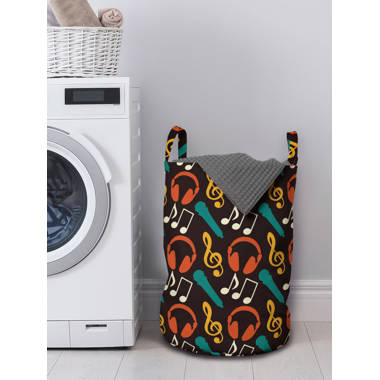In this image, we are inside a small laundry room. Prominently on the left-hand side is a front-loading white washing machine with a glass door, revealing some blue-colored clothes in the midst of washing. Atop the washer sits a white wicker basket containing neatly rolled-up towels in shades of pink and gray. The machine also features a small digital screen on the upper right side. To the right of the washing machine, positioned on the floor, is a cylindrical brown laundry hamper with a vibrant musical pattern. The hamper includes illustrations of green microphones, white musical notes, orange headphones, and a yellow treble clef. A gray towel drapes over the top, forming a V-shape. The hamper is equipped with two handles. The surroundings include a light gray wall with a white baseboard and small square white tiles covering the floor.